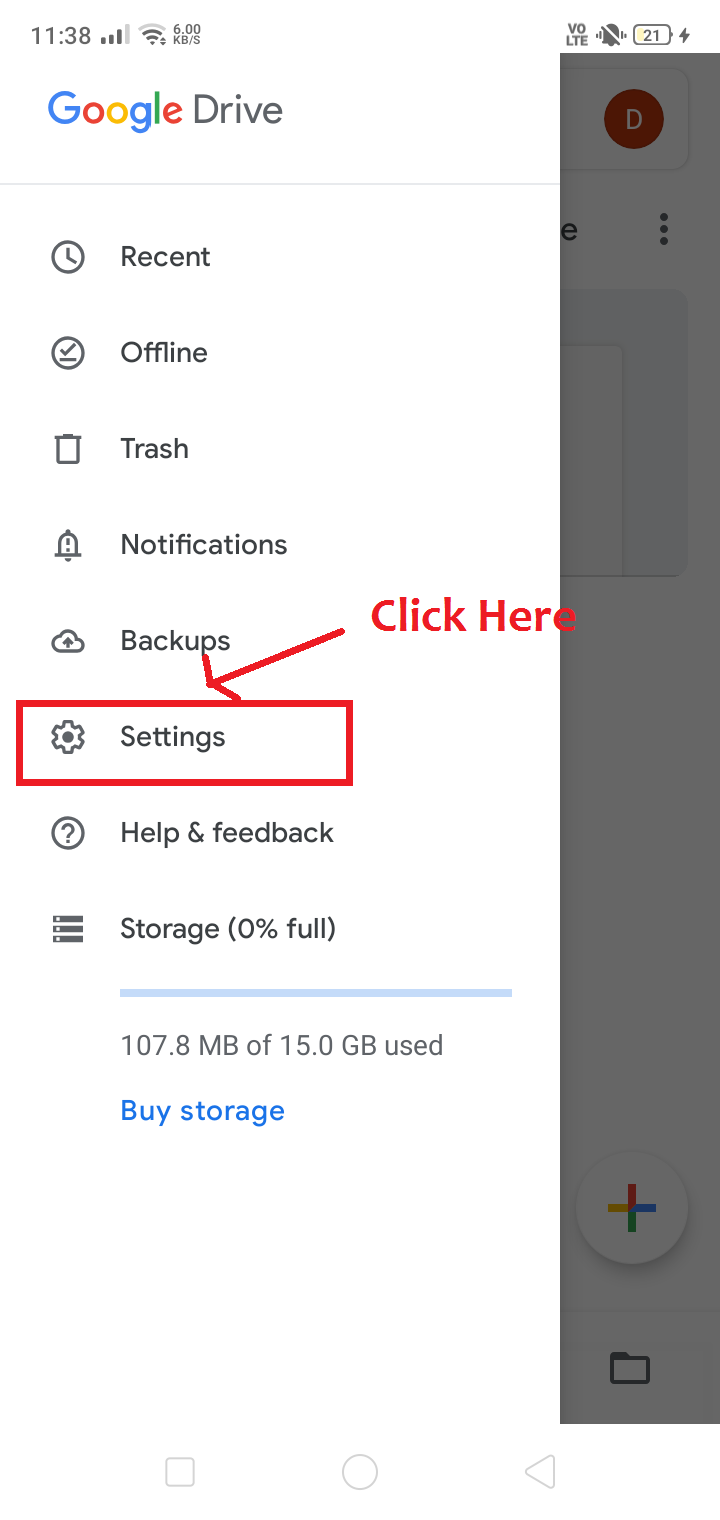The image is a cell phone screenshot displaying the Google Drive application. In the upper left corner, beneath the cell phone status icons, the Google Drive logo is visible. The main focus of the screenshot is a pull-out menu over a semi-transparent gray background, which reveals parts of the regular Google Drive interface underneath.

Prominently, a red box highlights the "Settings" option within the pull-out menu. The menu consists of seven options arranged vertically: 

1. Recent
2. Offline
3. Trash
4. Notifications
5. Backups
6. Settings
7. Help & Feedback

Below these menu options, there is an indicator showing that 0% of the storage is full. The white pull-out menu, contrasted against the gray backdrop, clearly organizes the user's navigation options within the Google Drive app.